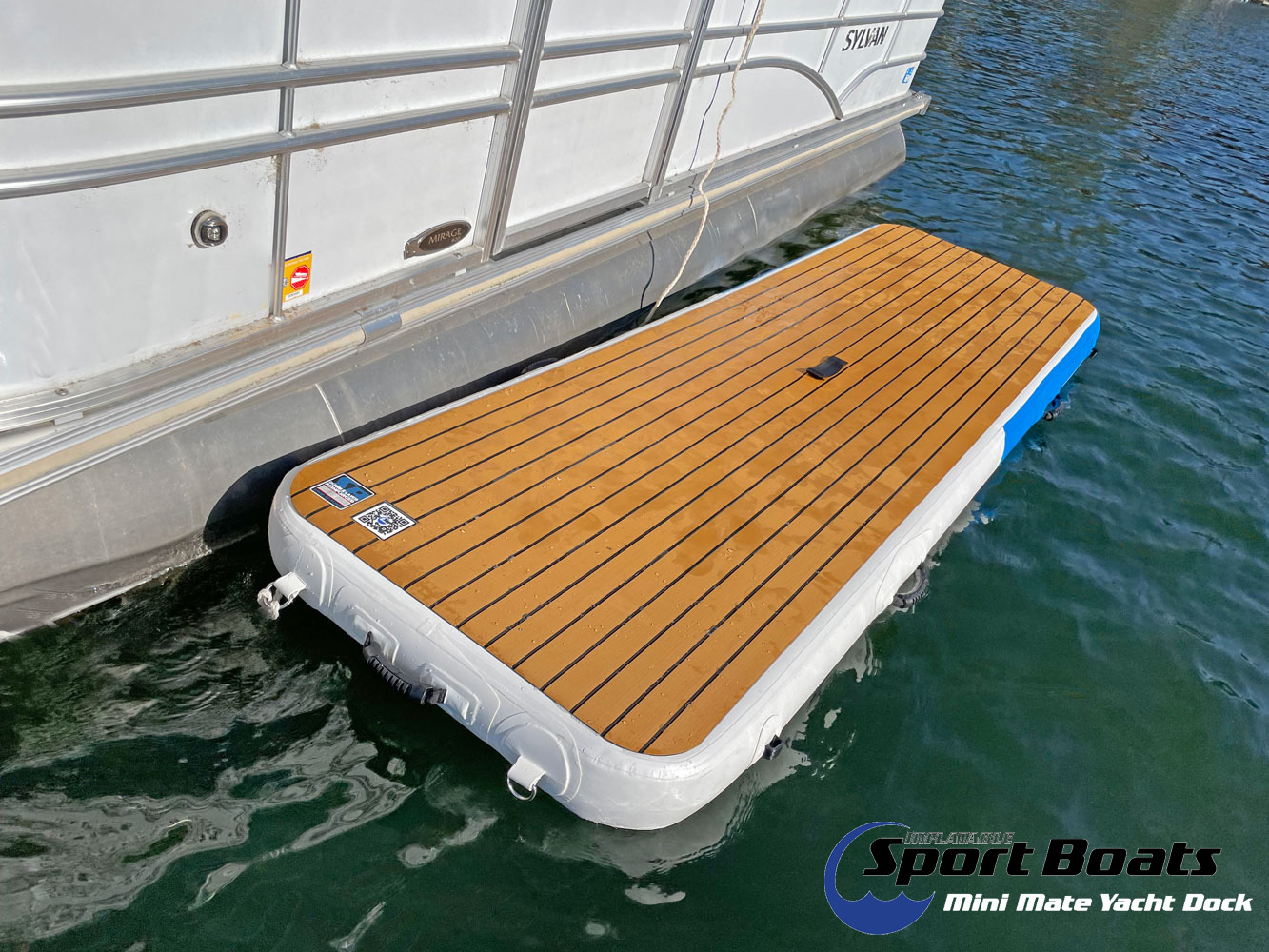This photo features a detailed view of a sleek pontoon boat with a pristine white body accented by silver framing. The boat is anchored in dark green waters, and tied securely to its side is a compact, inflatable dock. This dock has a visually deceptive top that mimics brown and black striped wood planks, but is actually made of durable plastic. It also has a sturdy black strap and a white rope tied to a small silver ring at the front of the pontoon. The sides of the dock are white with a black handle for easy maneuverability. In the bottom right corner of the dock, a logo stands out with its black text and blue wave accent, reading "SPORT BOATS" over smaller white text stating "MINIMATE YACHT DOCK." This descriptive caption highlights both the aesthetic and functional features of the pontoon boat and its accompanying inflatable dock.